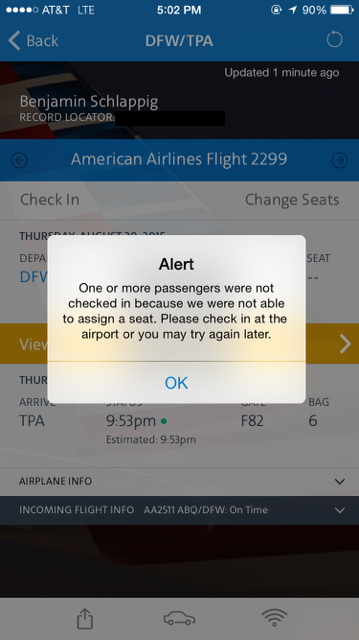A detailed screenshot of a mobile phone display features a central pop-up alert with a white background and black text that reads: "Alert: One or more passengers were not checked in because they were not able to assign a seat. Please check in at the airport or you may try again later." At the bottom of the pop-up, there is an "OK" button in blue, indicating it can be clicked.

The pop-up is slightly translucent, revealing a yellow band from the page behind it. The background image is greyed out, but several details are still visible. At the top, a blue band displays the time, 5:02 PM, along with AT&T LTE signal strength on the left and an 80% battery indicator on the right.

Below this, a black arrow and the text "DFW TRA" are seen, with a circle icon to the right and a black band underneath. The name "Benjamin Shapling" and a record locator appear on this black band, partially obscured by a grey marker attempting to conceal it. To the right, it indicates an update from "one minute ago."

Further down, another blue band shows "American Airlines flight 2299." The subsequent white band offers options to "Check-in" and "Change Seats." Partially visible yellow bands to either side of this segment hint at further information beneath the pop-up, such as "VIE" and a forward arrow on the right.

Additional details partially obscured by the pop-up include arrival information stated as "TRA 9:53 PM, F826, estimated 9:53 PM," followed by references to airplane info and an incoming flight with text too small to read clearly.

At the very bottom is a black banner, and below it, a grey strip contains an upload icon, a car icon, and a WiFi icon, all in black, indicating additional functions available on the screen.